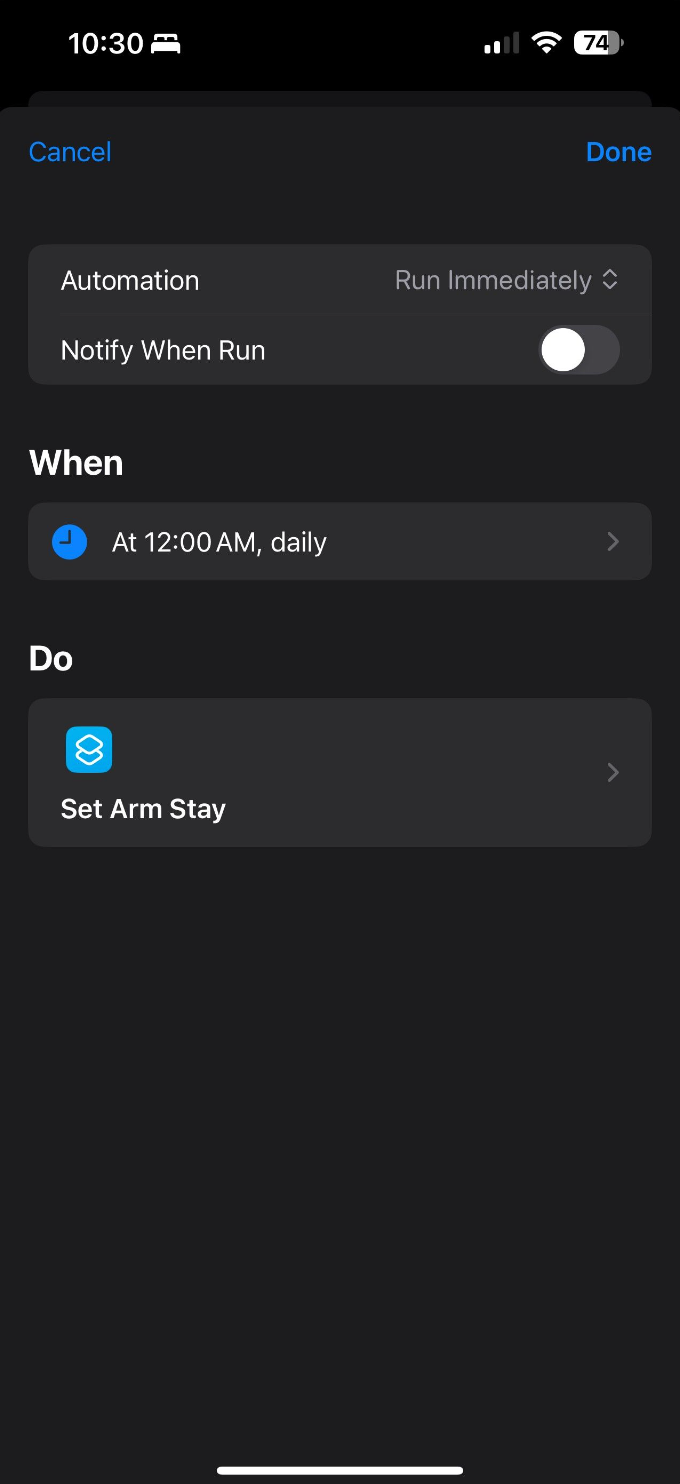The image showcases a user's cell phone screen, which features a black background. The time displayed in the upper left corner is 10:30. Adjacent to this, on the right, the phone shows a battery life of 74% and only 2 signal bars. Below these indicators, the screen displays the word "Cancel" in bright blue on the far left, balanced by "Done," also in bright blue, on the far right. Just beneath this row, there is a dark gray ribbon with the word "Automation" in bold white lettering, and opposite it, in light gray, it reads "Run Immediately."

Immediately below "Automation," there's a section labeled "Notify When Run," which is currently turned off. Under this, the bold white word "When" appears, followed by another gray ribbon containing a blue clock icon and the text "At 12 a.m." written in white, along with the specification "Daily." Continuing down, you see the word "Do" in bold white text, and underneath it, within yet another gray ribbon, the phrase "Set Arm Stay" is displayed. A notable light blue box is visible above this text.